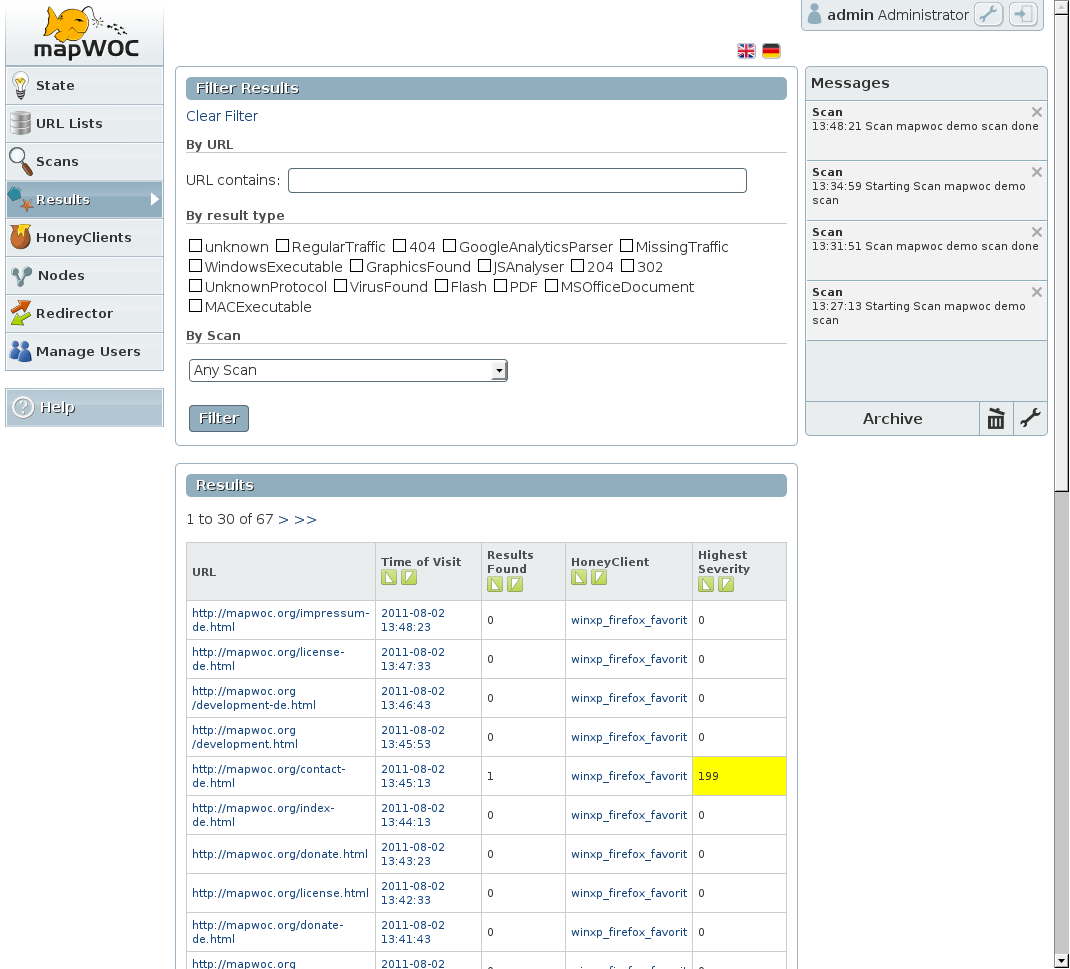This image is a snapshot of a user interface for a scanning and monitoring application. The main panel is titled "Map Walk" and features a visual representation of a large fish and several smaller fish. 

On the left side of the interface, there is a clickable menu with options labeled "State," "URL," "List," "Scans," "Results," "Honey Clients," "Nodes," "Redirector," and "Manage Users." Below this menu, there is a "Filter Results" section with various filtering options: "Clear Filter," "By URL," which allows filtering results that contain specific URLs, "By Result Type," "By Scan," with an option for "Any Scan," and a "Filter" button to apply these settings.

On the right-hand side, there is a messaging area displaying a list of scans, including titles like "Scan Map Walk," "Demo Scan Done," with a feature to archive these messages. 

The bottom part of the interface shows a results area. Here, the "Highest Severity" column indicates that one particular scan has flagged an issue with a severity score of 199, highlighted in a yellow box. All other entries show a severity score of zero, underscoring the significance of the single high-severity alert.